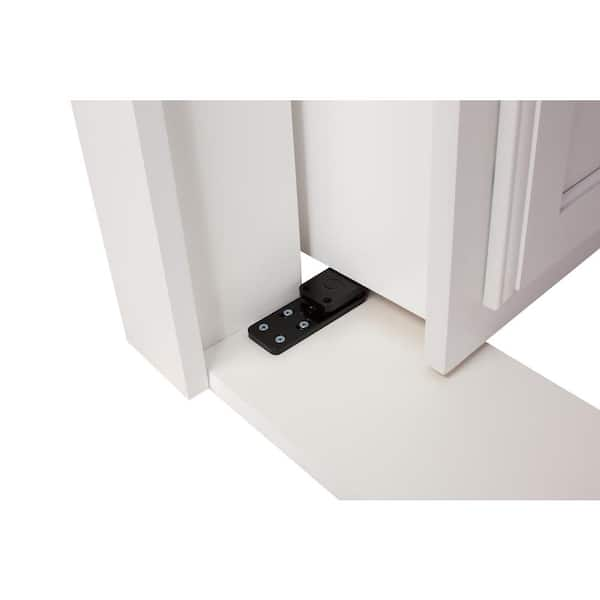This photograph features a detailed view of a door equipped with a Murphy-style mechanical key mechanism. The mechanism, constructed from black plastic components, consists of two main parts: one fixed section that is installed beneath the door, and another that functions as a sliding panel. The sliding mechanism can be moved and securely locked into place, ensuring the door can be opened only with a corresponding key. This setup is situated under a white cabinet-style door, with both the cabinet door and the nearby door jamb painted to match the surrounding decor. The sliding mechanism prominently features three gray circles, which serve as locking points that interlock with corresponding elements on the stationary black piece, securing the door effectively when engaged.